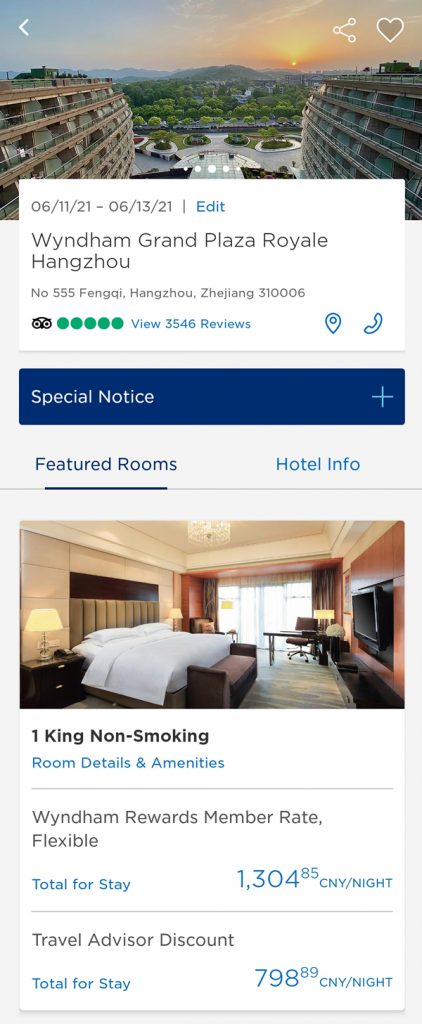This detailed image caption provides comprehensive information about a hotel, including its name, location, specific room details, and financial aspects:

---

Image Caption: 

The image depicts the luxurious Wyndham Grand Plaza Royale Hangzhou, a prominent hotel located in Hangzhou, Zhejiang, China, at 555 Fengqi Road (postal code 310006). This grandeur establishment boasts an impressive 3,546 reviews on TripAdvisor, reflecting its popularity and high standards among travelers.

The featured room showcased is a spacious King Non-Smoking Room, offering an array of amenities designed to ensure a comfortable stay. Wyndham rewards members can enjoy a flexible rate, with the total cost for the stay being 1,304.85 CNY (Chinese Yuan Renminbi), emphasizing the luxury and exclusivity of the accommodations. Alternatively, travel advisor discounts are available, reducing the total cost for the stay to 798.89 CNY per night, presenting a more budget-friendly option without compromising on quality.

The hotel's visual aesthetic includes a palette of colors such as white, blue, green, black, gray, brown, yellow, peach, rust, and varying shades of green and yellow, creating a vibrant and inviting atmosphere.

---

This caption integrates all the key details, providing a thorough and informative description of the hotel and its offerings.